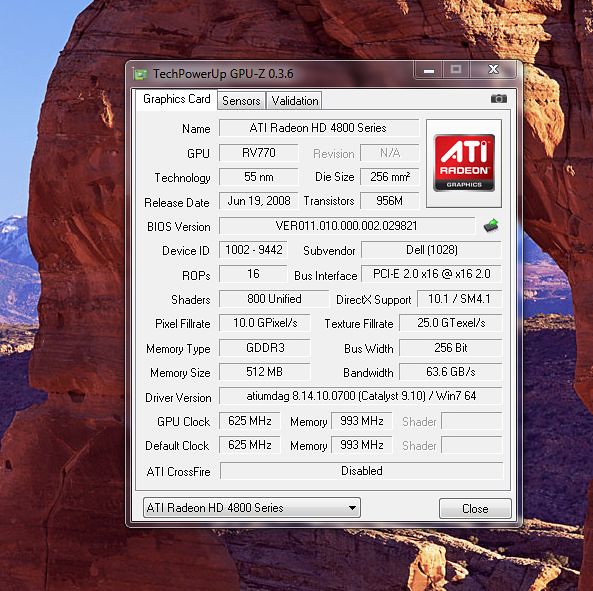The image depicts a computer screenshot featuring a dialog box of the TechPowerUp GPU-Z 0.3.6 program overlaying a scenic photograph of Arches National Park, recognizable by its iconic stone arches in the background. The dialog box, aligned with the top of the screen, displays tabs labeled "Graphics Card," "Sensors," and "Validation," with the "Graphics Card" tab currently open. It provides detailed specifications of an ATI Radeon HD 4800 Series graphics card, including fields such as GPU (RV770), Technology (55nm), and Release Date (June 19, 2008). Additionally, it lists Die Size (256mm²), Transistors (956M), and BIOS Version (VER 011.010.000.002.029821). Other details include Device ID (1002-99442), Subvendor (Dell 1028), ROP (16), and various performance metrics such as Bus Interface (PCI-E 2.0 x16 @ x16 2.0), Shaders (800 unified), DirectX Support (10.1/SM 4.1), Pixel Fillrate (10.0 GPixel/s), Texture Fillrate (25.0 GTexel/s), and Memory Type (GDDR3). It notes a Memory Size of 512MB, Bandwidth of 63.6 GB/s, Driver Version (ATI UMDAG 8.14.10.0700 with Catalyst 9.10), GPU Clock (625 MHz), Memory Clock (993 MHz), alongside default clock speeds, and the status of ATI CrossFire (disabled). Positioned at the bottom left is a button labeled "ATI Radeon HD 4800 Series" with a dropdown arrow, while the close button is located at the bottom right of the dialog box. The top of the window features the program's name and typical window control buttons to minimize, maximize, or close the window. The ATI logo, a red background with white letters, is visible at the top right corner of the window.